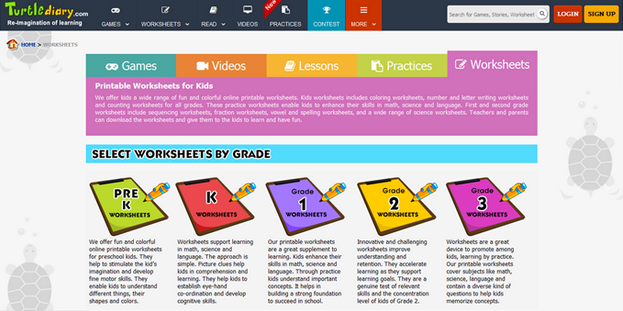This webpage screenshot is from "turtlediary.com," a platform dedicated to providing educational activities and printable worksheets for elementary school children. The top navigation menu features icons for various resources, including games, worksheets, reading materials, videos, practice exercises, contests, and more. On the far right, there are options to search, log in, or sign up.

Beneath the main navigation, there's a secondary bar that repeats categories such as games, videos, lessons, practice exercises, and worksheets. The focus of the screenshot appears to be on the "Worksheets" section, as indicated by the highlighted category and the accompanying explanation "Printable Worksheets for Kids," which suggests that hovering over the word provides additional information.

A prominent blue bar invites users to "Select Worksheets by Grade," listing options for Pre-K, Kindergarten, 1st Grade, 2nd Grade, and 3rd Grade. Each grade level is represented by a colorful, themed worksheet icon:
- Pre-K features a green worksheet with a small pen hovering over it,
- Kindergarten has a red worksheet,
- 1st Grade is represented by a purple worksheet,
- 2nd Grade is yellow,
- 3rd Grade is depicted with a dark pink worksheet.

Under each grade category, there's a brief description. For instance, the Pre-K section explains, "We offer fun and colorful online printable worksheets for preschool kids. They help to stimulate the kids' imagination and develop fine motor skills. They enable kids to understand different things, their shapes, and colors."

The webpage has a colorful design with child-friendly elements, such as small turtles adorning the sides, reinforcing its educational focus for young children.